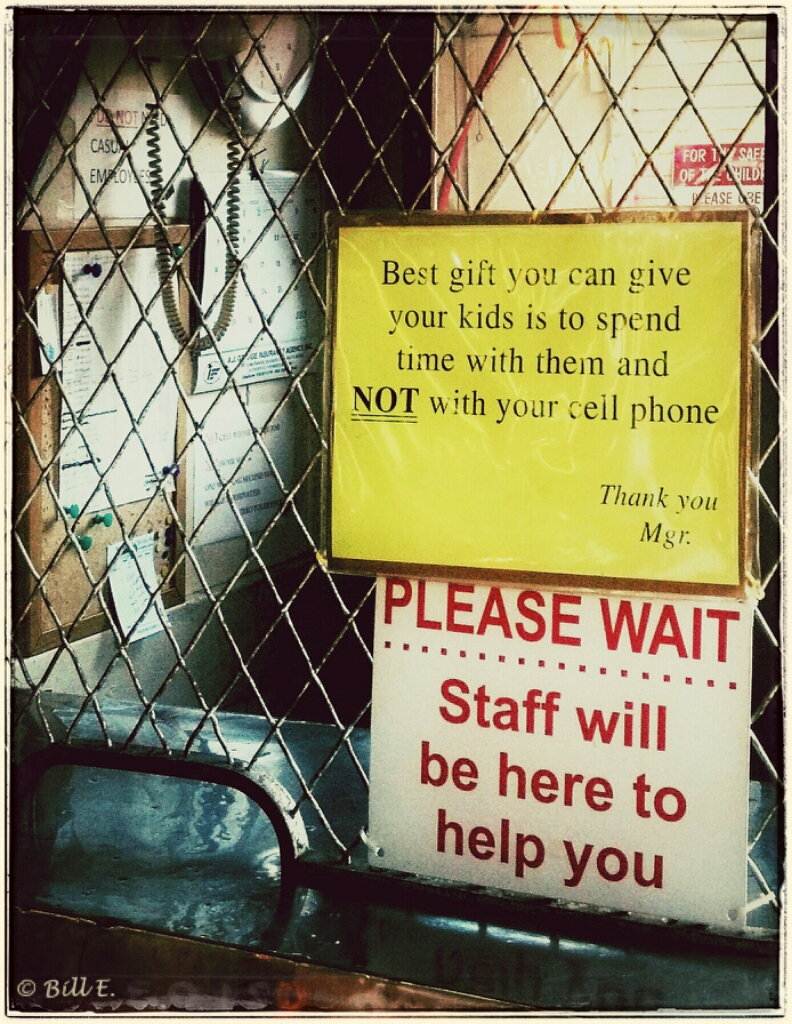The photo depicts the interior of a dated office, specifically a ticket booth or service counter setup. The scene is dominated by a black counter topped by a mesh frame with an opening for transactions. This wired divider is prominently featured with two signs: a yellow sign with black text reading, "The best gift you can give your kids is to spend time with them and not with your cell phone. Thank you, MGR," and directly below it, a slightly smaller white sign with red text stating, "Please wait, staff will be here to help you." The backdrop includes a dimly lit bulletin board cluttered with papers and a coiled telephone cord extending from a speaker, suggesting a utilitarian and somewhat dated office environment. The counter itself reflects a turquoise hue, and the office background is painted in a light blue and off-white color scheme, enhancing the sense of an older, well-worn space.